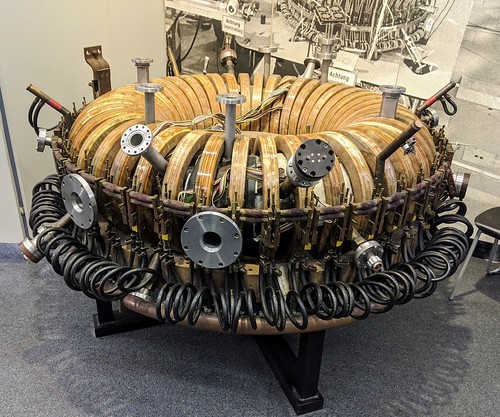This rectangular photograph showcases a complex, round machinery-like device prominently in the foreground, possibly displayed in a museum setting. The apparatus has a distinctive donut shape comprised of concentric, wooden ring-like segments forming its structure. A combination of pipes, pistons, and metal bars project from various points around the device, contributing to its intricate appearance. The base of the unit features loops of coiled black hoses or wires, accentuating its detailed design. The device is mounted on a black metal stand, though it's unclear whether the stand is integral to the apparatus or merely for display purposes. In the background, a black and white illustration of the device provides additional context, resembling a technical drawing of the same object. The scene is set against a gray carpeted floor, emphasizing the polished and curated presentation of what may either be an antique machinery replica or an elaborate art piece.